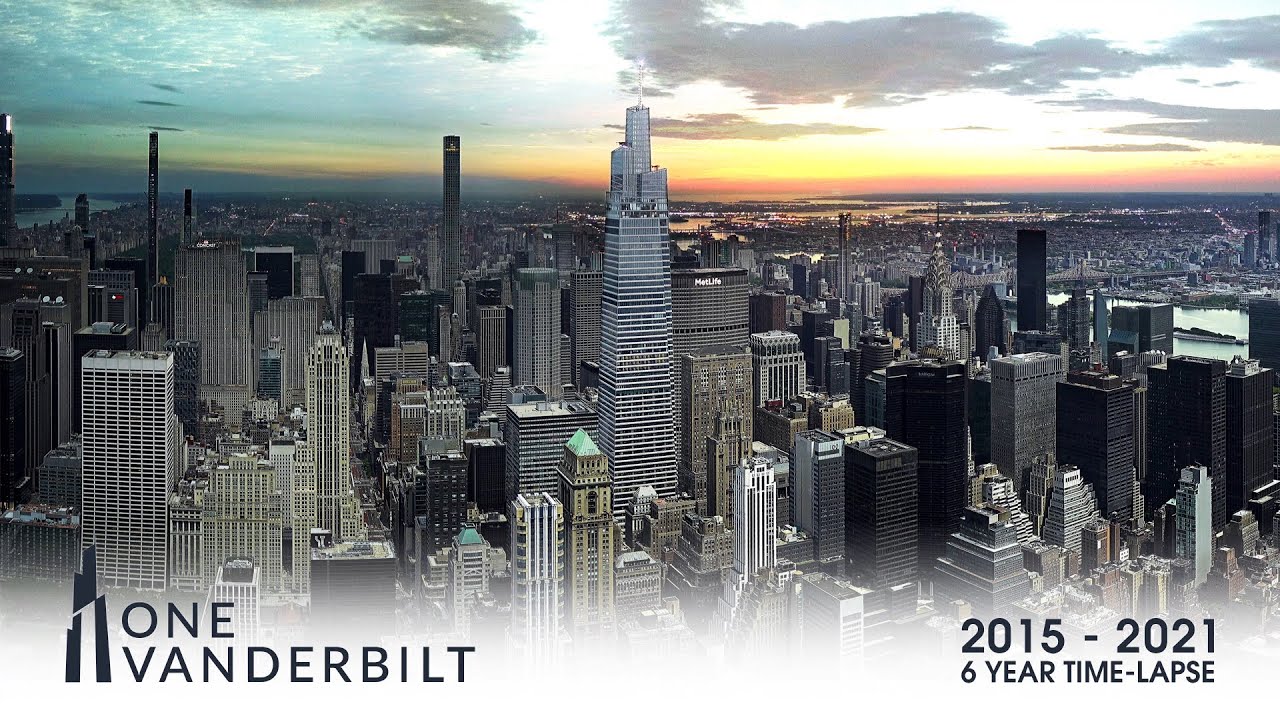This image depicts a sprawling cityscape, likely representing New York or Manhattan, captured either at dawn or dusk, highlighted by a vibrant sky blending cyan, orange, and red hues. Dominating the center of the photograph is the prominent One Vanderbilt skyscraper, identifiable by the three distinct pillars of varying heights at its top. The surrounding city is filled with numerous other skyscrapers in shades of gray, beige, and white, with some featuring cyan roofs. Located in the bottom left corner is the logo and black text reading "One Vanderbilt," set against a white backdrop, indicating the image likely belongs to a montage or video. In the bottom right corner, text reads "2015-2021 six-year time lapse," suggesting this image is part of a series documenting the construction or transformation of the city over six years. The scene is completed by a serene sunset or sunrise, casting a warm glow over the expansive, modern metropolis.